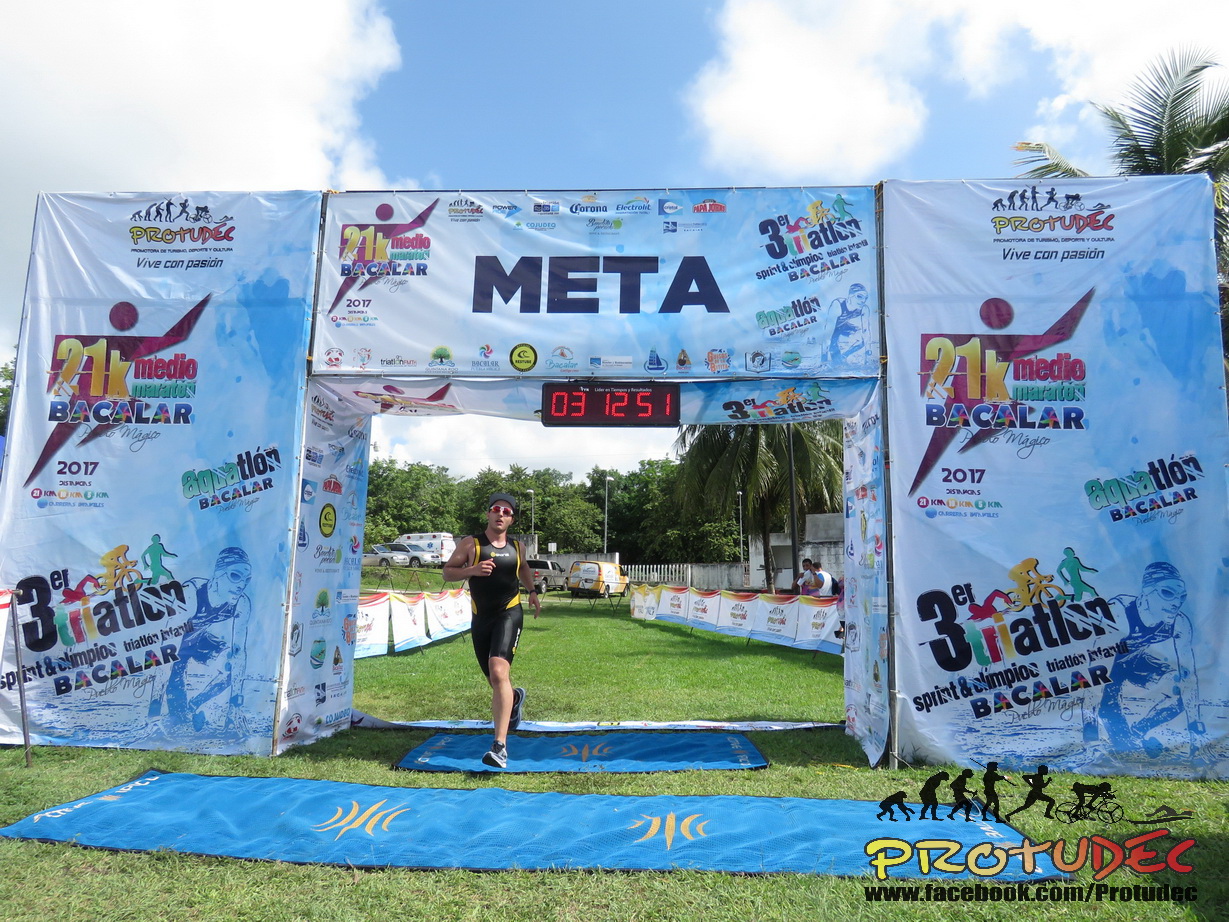The photograph captures a lively outdoor scene on a bright, partly cloudy day in a tropical environment. Dominating the right-hand side of the image are tall, swaying palm trees, adding to the serene ambiance. Featured prominently at the foreground is a man dressed in a black jogger's outfit, energetically crossing a finish line. This finish line is an archway made up of cardboard and festooned with various banners, among them a notable one that reads "21K Bacalar" and another that states "META" in bold blue font. Above the runner's head is a digital scoreboard displaying the time "3:12:51." Below the archway, two blue carpets lay sprawled out, guiding the participants. Additionally, there is an intriguing illustration on the right side of the image, depicting the evolution from monkey to a human in various stages of running and biking, accompanied by the logo and website "ProTutor www.facebook.com." The event appears to be part of a three-year triathlon series, potentially sponsored by Baccalaureate, ProTutor, and MEDA, and is possibly dated 2017.